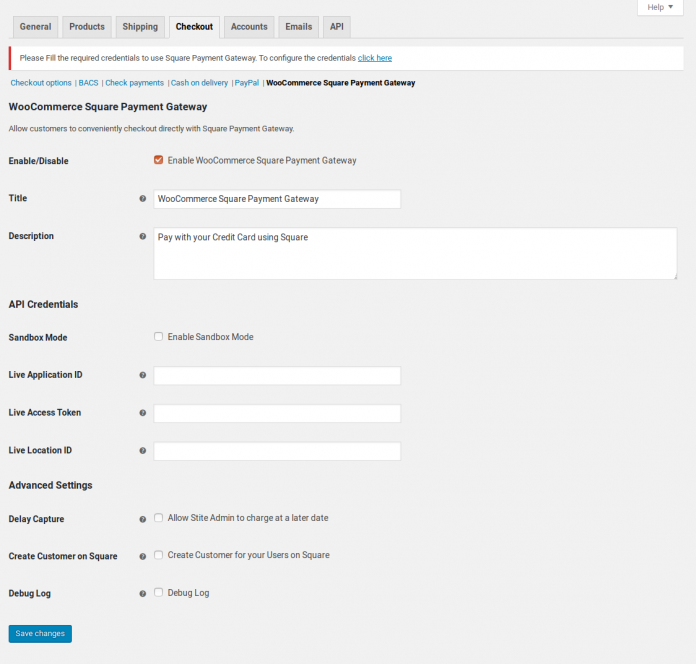The screenshot showcases a webpage dedicated to setting up the WooCommerce Square Payment Gateway. The overall theme consists of a muted gray background at the top, providing a neat contrast to the various tabs present. These tabs include options such as "General," "Products," "Shipping," "Checkout," "Accounts," "Emails," and "API." 

Beneath these tabs, the page title "WooCommerce Square Payment Gateway" prominently identifies the section's purpose. Positioned at the top is a bar with a prominent red sidebar that contains a notice reading, "Please fill the required credentials to use Square Payment Gateway. To configure the credentials, click here." 

This message implies that the user must input necessary authentication details to fully enable the payment gateway. Judging by the context, it appears that the user is in the midst of setting up the Square Payment Gateway to facilitate transactions for their online store or other sales platform.